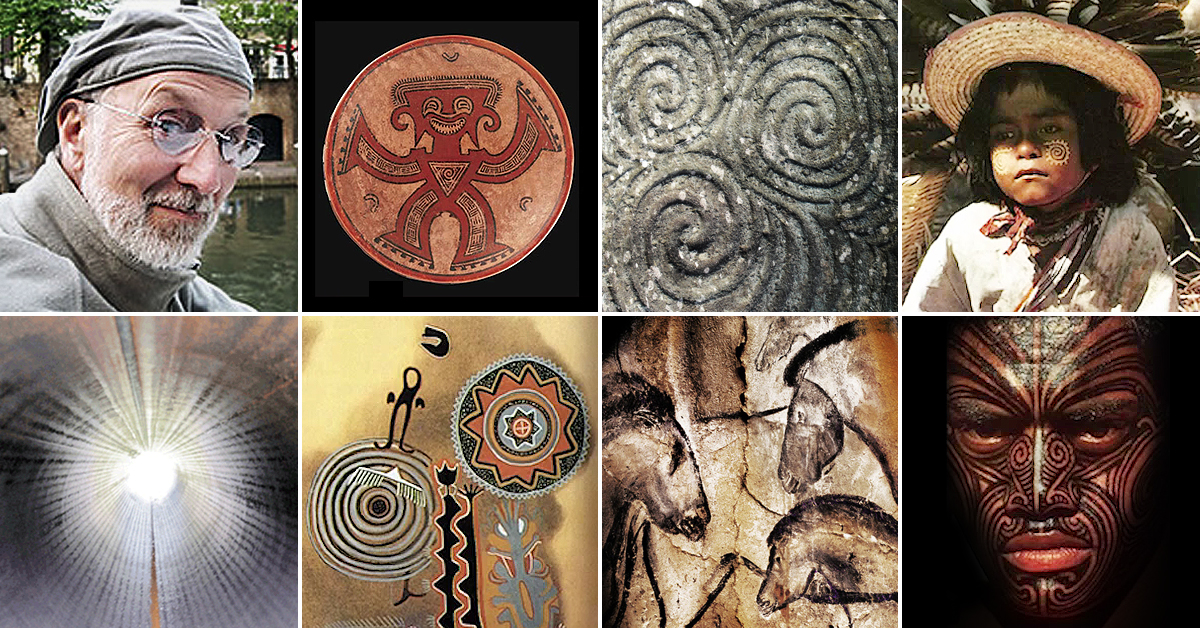The image is a collage of eight photographs arranged in two rows. In the top left corner, there's an older gentleman with a grey beard, small round glasses, and a slouchy artists' beret turned backwards. He is dressed in a grey fleece jacket and appears in a poolside setting with water in the background. Next to him, there's a red circular tribal artifact, possibly Incan or Mexican, depicting a person with raised arms, a triangular center, and spread legs. This is followed by a photograph of silver spirals, reminiscent of rock formations or sculptures. The fourth image in the top row is of a young child with face paint, wearing a hat and a bandana around the neck, giving a thoughtful expression.

In the bottom row, directly beneath the child, there is a drawing of a face adorned with Maori-style tattoos, characterized by intricate swirls covering the adult's complexion. Beside this, to the right, is a depiction of three horses from a cave drawing or rock wall, resembling ancient hieroglyphics. Next to the horses is a colorful design featuring circular patterns, potentially representing traditional Mexican or Incan art with possible symbolic meanings. The final image in the bottom right corner is of a radiant sunburst design, emitting beams of light from its center, which could be interpreted as a pottery piece or a painting.

Overall, the collage combines a mix of cultural and archaeological imagery with portraits, highlighting the diversity of human expression through art and tradition.